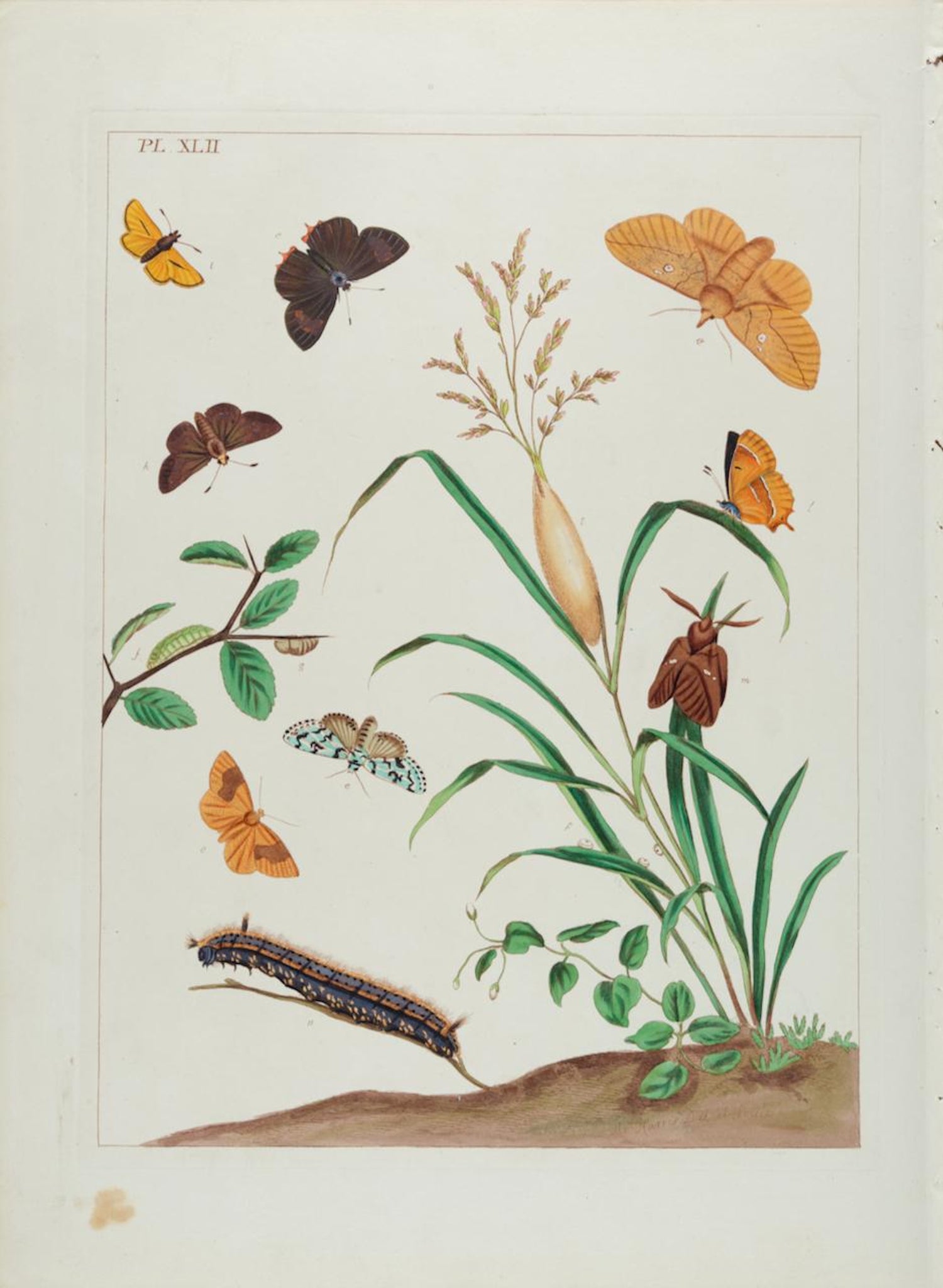This detailed nature print, which resembles a painting or a finely drawn illustration, showcases a rich variety of butterflies, moths, and caterpillars amidst a natural setting. At the top, the image is labeled "PL. XL, II," with an obscure signature in the bottom right corner. The scene includes an assortment of insects: yellow and black moss-like butterflies, blue and yellow-winged butterflies, and various moths with distinctive patterns. On the bottom right, a caterpillar is perched on a branch, which extends from a plant with thin green leaves. Another branch enters from the left side, hosting two caterpillars—one brown and one green. The background features dirt with minimal vegetation, save for a single plant with a few leaves. Colors in this composition include shades of green, brown, orange, beige, light blue, off-white, and dark brown, adding to the natural and diverse appearance of the scene. The illustration captures the intricate details and various stages in the lifecycle of these insects, set against a backdrop of leaves and sparse vegetation growing out of brown earth.